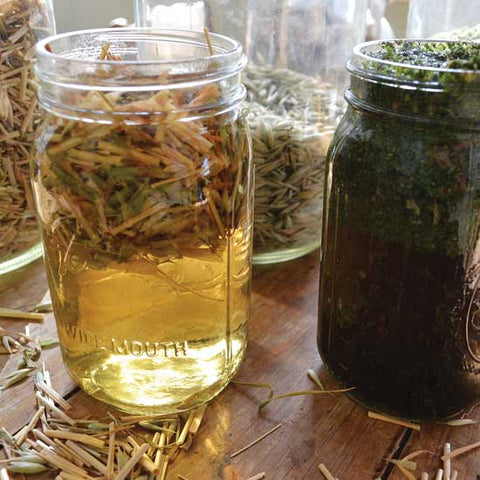The image features four mason-style jars, prominently displayed on a wooden, picnic-like table with visible slats. On the far left, there is a jar filled with light-colored dried vegetation, possibly grains or herbs. Next to it, in full view, is another jar with a similar dried substance occupying the upper half, while the bottom half is filled with a weak yellow liquid, perhaps resembling apple juice. To the right, a jar partially visible in the frame is completely filled with dark green chopped vegetation, which might be similar to spinach. Behind these jars, a larger jar partially seen is also filled with the light-colored dried material. The background includes more jars or pitchers containing plant material, contributing to a color palette that ranges from green and brown to yellow and white.